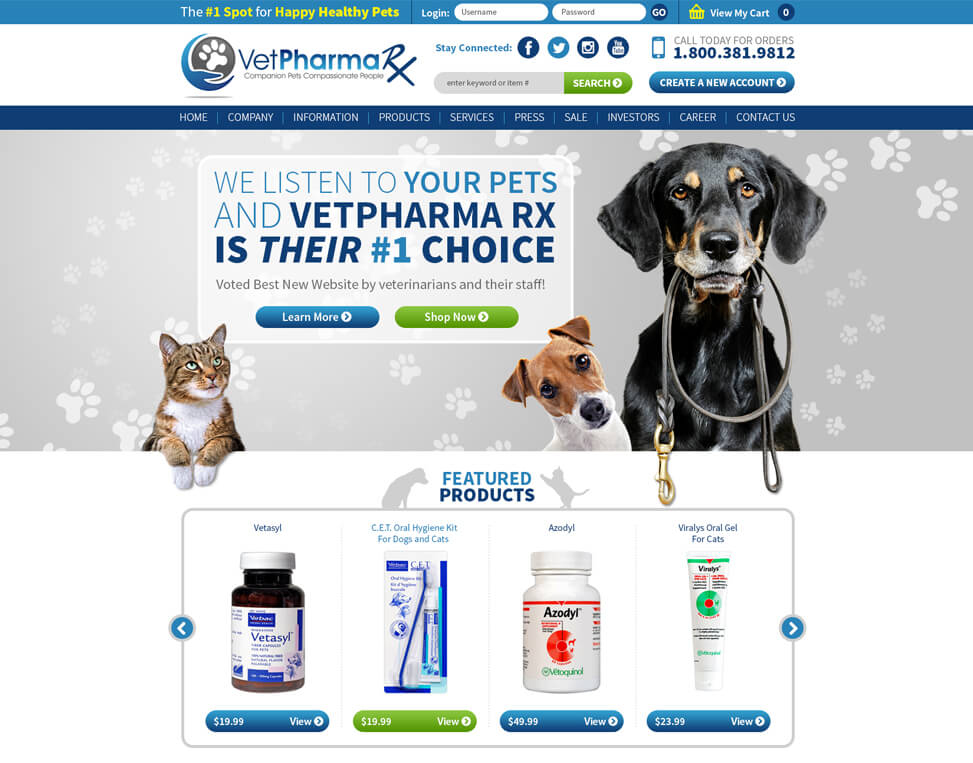In the image, we observe an online sign-in page for a company called Vet Pharma RX. The Vet Pharma RX logo is prominently displayed in the top left corner, with a tagline above it that reads, "The number one spot for happy, healthy pets." Central to the image is a login box that prompts users to enter their username and password, accompanied by a "Go" button. To the right of the login box is a small house icon labeled "View my cart."

Adjacent to the login section, on the right, we find several social media icons encouraging users to "Stay connected" via Facebook, Twitter, and Instagram. There's also a phone icon, along with the phrase "Call today for orders," followed by the number 1-800-381-9812. Below this, there's a search bar where users can enter keywords or item names, paired with a green "Search" button. Further to the right, a blue button invites users to "Create a new account."

Towards the bottom of the image, there's a navigational section featuring linkable instructions for "Home," "Company," "Information," "Products," "Services," "Press," "Sale," "Investors," "Career," and "Contact Us." A highlighted phrase declares, "We listen to your pets and Vet Pharma RX is their number one choice, voted best new website by veterinarians and their staff," along with "Learn more" and "Shop now" buttons.

To the left of the central marketing piece, a small cat with its paws up is visible. On the right side, there is a small dog and a larger black dog holding a black leash with a gold buckle in its mouth. Below the dogs, the image showcases four products under the heading "Featured Products," listed from left to right: Vita Sal, an Oral Hygiene Kit for dogs and cats, Exedil, and Viralis Oral Gel for cats, each with their respective prices displayed.